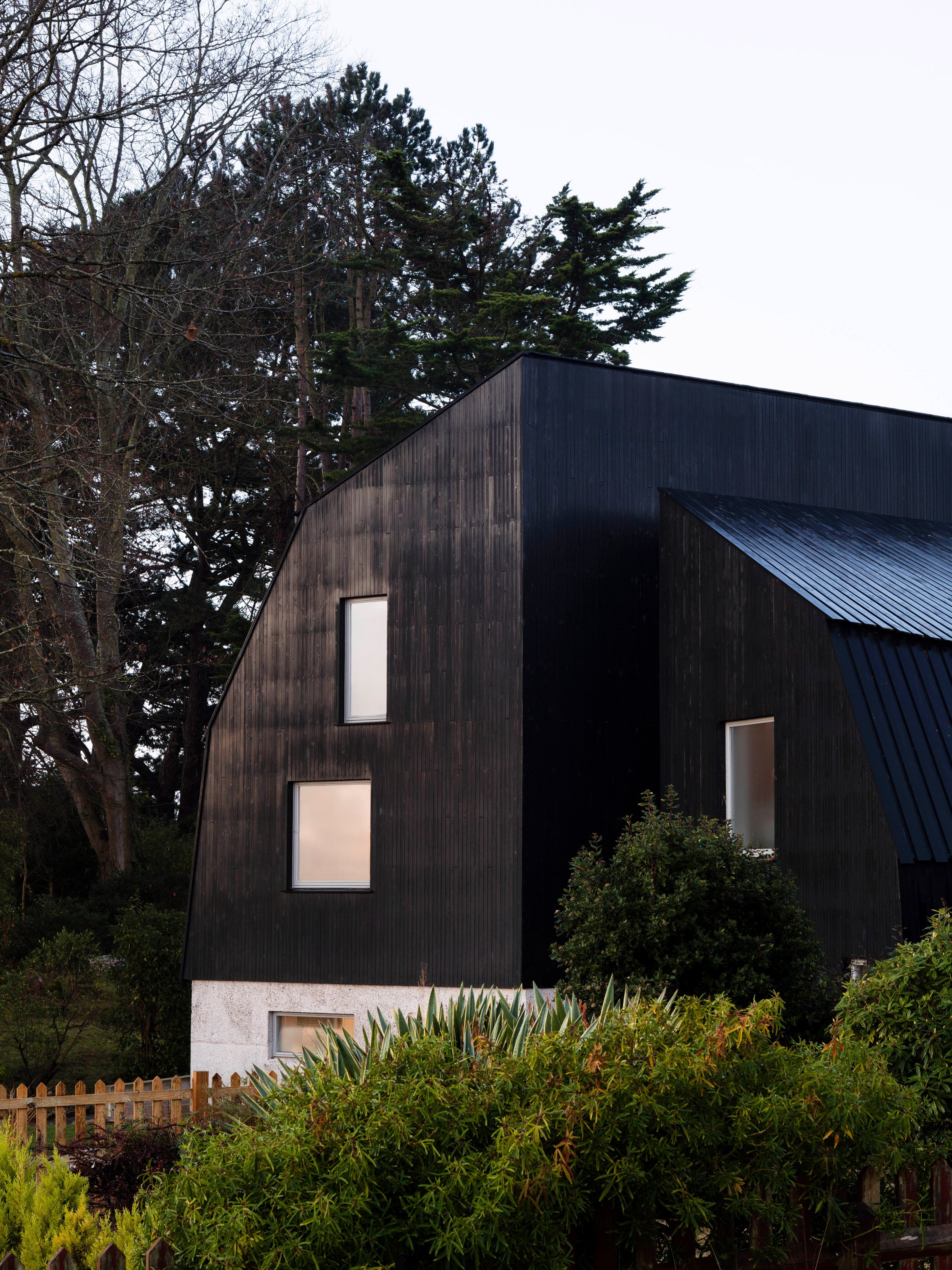The photograph depicts the side of a modern, industrial-type building with a distinct architectural style. The structure features a striking, almost black exterior wood paneling that transitions into a white, cement-like base. The side of the building includes frosted windows—two on the left section and one on a protruding middle section—which obscure any view inside. Below the windows on the left is a small rectangular window embedded in the white base.

In the foreground, there is a well-manicured line of green bushes extending from the left to the right, intersected by a brown wooden fence that runs diagonally from the bottom left towards the middle of the image. Just in front of the building, on the right side, stands a larger bush or small tree with green leaves, adding to the semi-wild but maintained aesthetic.

In the background, a variety of trees, some with green leaves and others bare, create a natural backdrop. The larger trees rise above the roofline, their tops visible against a gray, cloudy sky that blankets the scene, suggesting it is possibly a cloudy day. The overall ambiance balances between modern construction and natural elements, harmoniously blending the built environment with its green, slightly untamed surroundings.